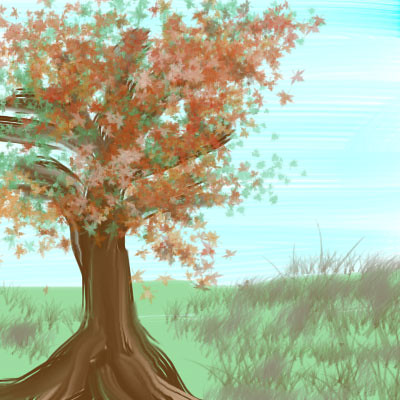This image depicts a vibrant watercolor painting of a large tree, prominently positioned on the left side of the canvas. The tree's thick trunk is a deep, rich brown with highlights that add depth and texture. The foliage displays an array of autumnal hues, transitioning between red, orange, and brown, suggesting a seasonal change. Some leaves appear to be falling, adding a dynamic quality to the scene. The sky above is characterized by thick brush strokes, blending bright blue and white, and showing streaks of clouds that create a sense of movement. The background may hint at the presence of water due to the perspective and colors used. Below, the field is lush and green, with variations in the grass height and color, interspersed with small bushes, weeds, and even some tall, brown grass. The painting overall is highly detailed and vividly colorful, capturing the essence of a serene, transitional moment in nature.